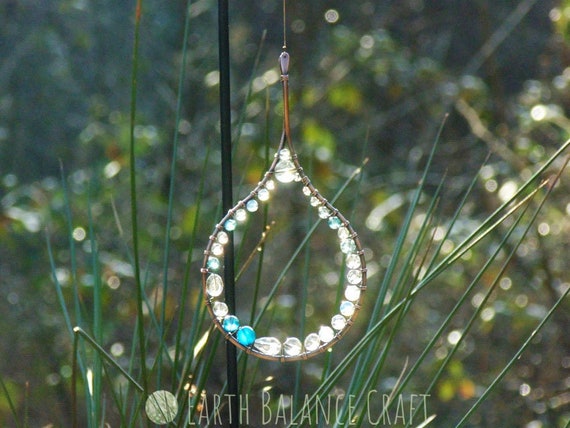The image depicts an outdoor scene featuring a handcrafted hanging decoration suspended from a black metal rod. The ornament is intricately designed with a copper or metal wire frame shaped like an elongated water drop or oval loop. Inside the wire frame, there is an arrangement of variously sized crystals, which include a mix of clear, blue, and some with a faint pink tint. At the top of the loop sits a prominent large crystal, which transitions into smaller stones towards the middle and then larger ones again near the bottom. Blue and clear crystals are interspersed throughout the loop, creating a visually appealing pattern. The background shows a grassy area with bushes and shrubs, illuminated by sunlight. Below the decorative piece, the words "Earth Balance Craft" are visible as a semi-transparent watermark in capital letters.